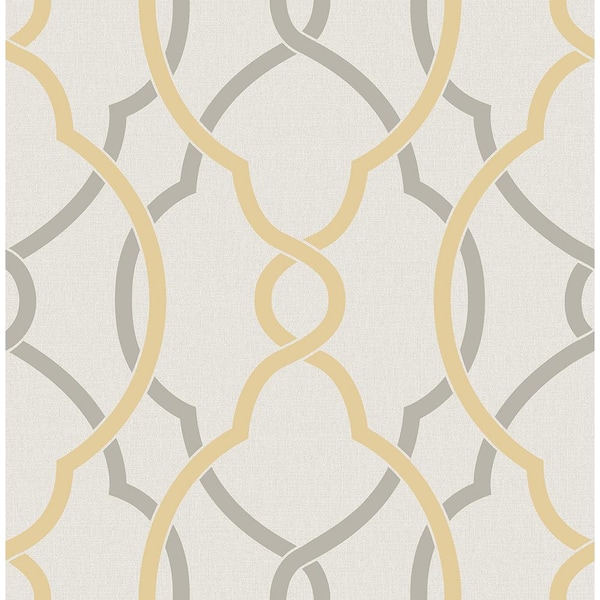The image depicts a detailed pattern consisting of four primary curved lines, both in beige and gold hues, that intersect at two central points. These main lines are overlayed on a textured light gray or light beige background with a linen-like appearance. Behind these dominant lines, there are four additional curved lines in a gray or silver color that emerge from the edges of the image, creating a layered effect. The overall design gives the impression of an intricate wallpaper pattern, possibly a digital representation, with a somewhat formal, vintage aesthetic. The lines and curves are arranged in a mirrored fashion, with gold lines forming wishbone-like shapes that entwine with the silver behind them. The pattern suggests a balanced yet elaborate design, suitable for a formal living room, reminiscent of decor popular in the 2010s.